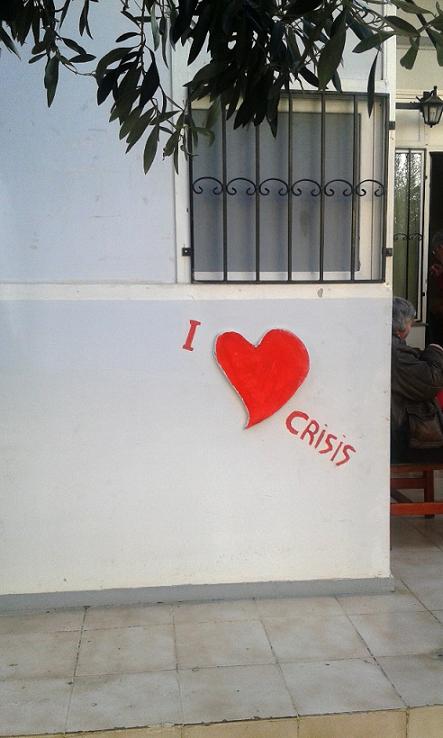This photograph captures a rectangular building, taller than it is wide, presumed to be either a house or an apartment block. The focal point is a white wall that features a square window adorned with black security bars. Above the window, there is a light fixture. The window also reflects some trees, indicating the outdoor setting. A message is prominently displayed on the lower portion of the wall, crafted from cut-out cardboard letters in red, forming the phrase "I ♥ Crisis." The wall shows signs of wear with chipping white paint. To the right of this message, partially visible, is an elderly person with gray hair sitting on a red bench or chair, suggesting they might be a resident or a visitor. The ground is made up of cement blocks arranged in a square pattern, and some green tree leaves are visible in the upper part of the image, hinting at a tree overhead. The steps leading up to the property appear old and in need of maintenance.